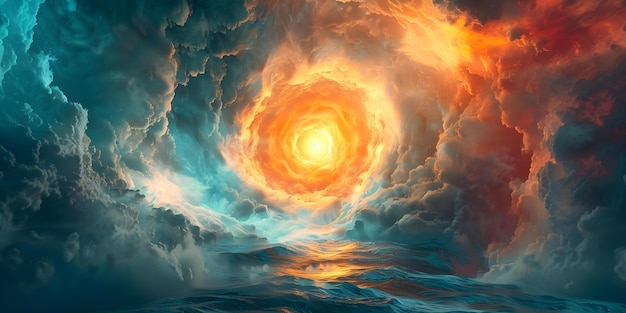This abstract painting captures the dramatic clash between the sun and stormy clouds swirling around it. At the center lies a radiant sun, depicted as a bright light source, serving as the focal point of the artwork. Encircling the sun are turbulent clouds that resemble billowing red and yellow smoke, gradually transitioning into darker hues. On the right-hand side, the colors deepen into shades of red and gray, creating a sense of foreboding. Conversely, the left-hand side features a mix of turquoise, black, and white clouds, swirling in a dynamic motion, adding to the stormy atmosphere. The overall composition evokes the eye of a storm, as if seen on the horizon, with the entire scene rendered in a distinctly artistic style rather than a photorealistic one. The painting exudes intensity and movement, drawing viewers into the tempestuous interplay of light and dark elements.